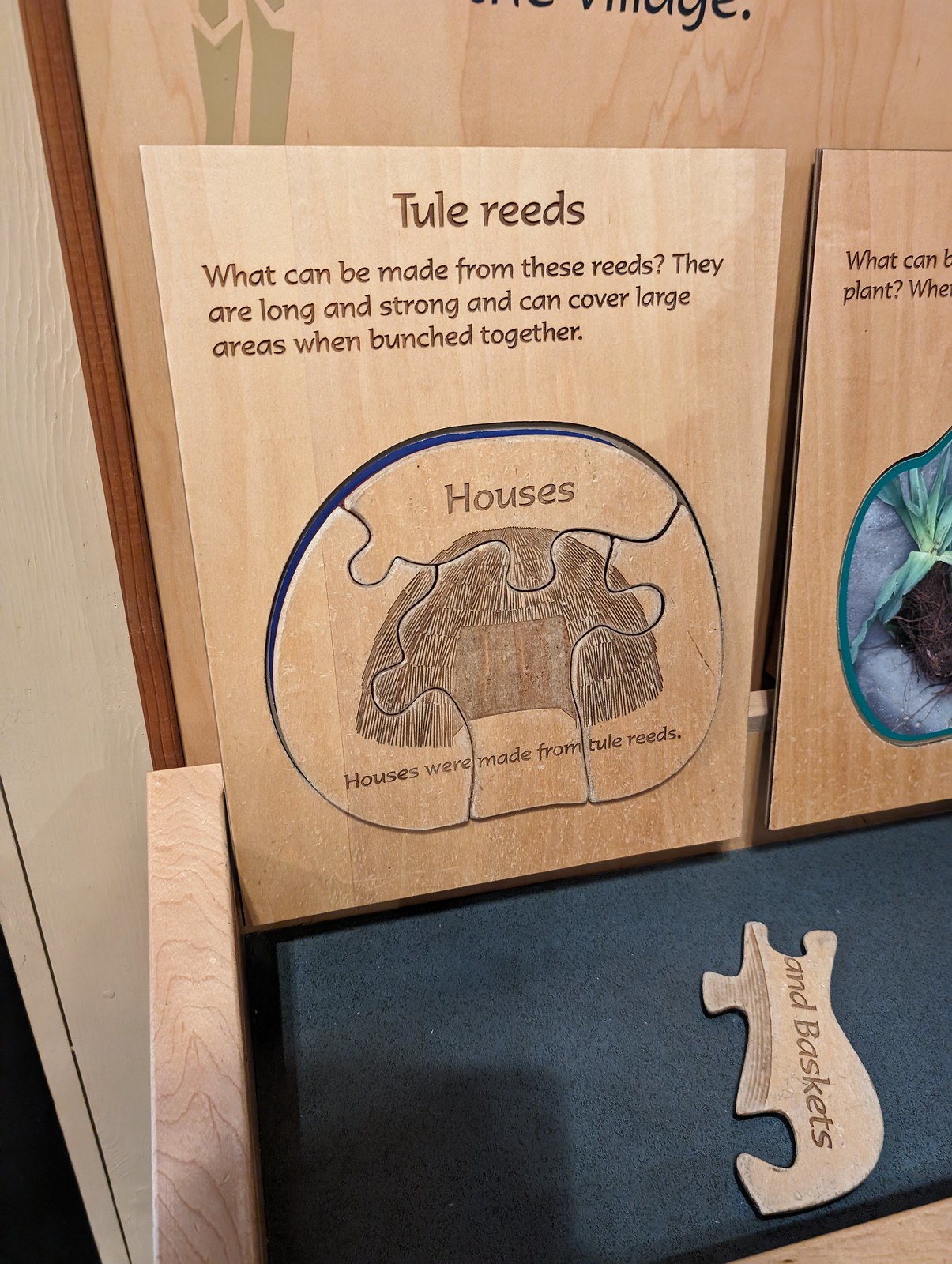This detailed color photograph captures a horizontally aligned educational display, likely found in a nature center or an educational space, featuring wooden panels and puzzle pieces on a finely sanded tan wood background. The image prominently displays two standing wood panels, one on the left and one partially visible on the right. The left panel is headed by the text "Tool Reeds" in a dark color, which appears to be written in a papyrus font. Below this header, the text reads: "What can be made from these reeds? They are long and strong and can cover large areas when bunched together," aligned to the left. 

Beneath this explanatory text, there's an oval-shaped cut-out puzzle with four pieces, completed to depict a thatched roof structure labeled "houses." The caption below the structure states, "Houses were made from tool reeds." The right panel features a beautiful blue design with intricate detailing and partially visible text, including the phrases "what can," "plant?" and other obscured words. 

Both panels are elevated on a surface covered in dark blue fabric, and in the foreground, there is a visible puzzle piece featuring the word "baskets." A shadow from a tan wooden piece is cast onto the navy blue fabric, adding depth to the composition. Additional elements such as a paler wooden panel and a small black triangle can be seen on the left, hinting at more interactive aspects of the display. The overall presentation gives an impression of carefully crafted educational material, possibly used in a nature-focused or early childhood learning environment.